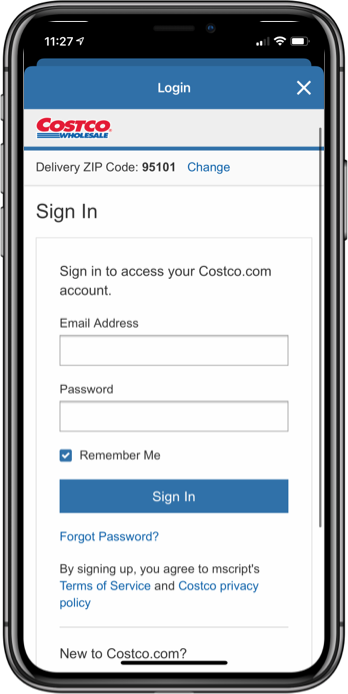A detailed screenshot of a phone displaying the Costco website's login page. The image features a phone border that includes visible buttons on the sides and the front camera. The phone's status bar indicates the time is 11:27. Location services are enabled, there are two bars of signal strength, Wi-Fi is connected, and the battery level is between 80% and 90%.

At the top of the screenshot, a blue banner with white text prompts the user to log in. Directly beneath this, the Costco logo is situated on the left side, followed by a section stating the delivery zip code as "95101." A blue button labeled "Change" is next to this zip code information. Below, there is a login form consisting of fields for entering an email address and password. A checked checkbox labeled "Remember Me" is also visible.

Underneath the login fields, there is a prominent blue "Sign In" button with white text. Below this, there is blue text stating "Forgot Password?" Additionally, a note at the bottom mentions that by signing up, users agree to the "Terms of Service" and "Costco Privacy Policy," with these links highlighted in blue text. Further down, a question reads: "New to Costco.com?"

The image also includes the iPhone's home bar, indicating that this screenshot was taken on an Apple device. 

This caption provides a thorough description of the Costco website login page as seen on a mobile device, detailing both the webpage elements and the phone's interface.